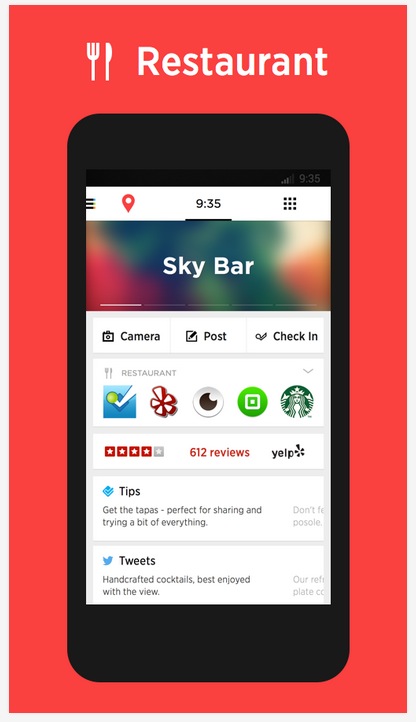The image displays a vibrant advertisement with a bright red background. At the top center, the word "Restaurant" is prominently displayed in white text, accompanied by a small symbol featuring a fork and knife. Below this, an illustrated black phone is depicted. On the phone's screen, at the top, it reads "9:35," followed by "Sky Bar" in white text.

The phone interface shows three distinctive buttons: 
- The left button is labeled "Camera," featuring a camera icon. 
- The middle button is labeled "Post," accompanied by a small note and pencil icon.
- The right button is labeled "Check-in."

Further down, the screen repeats the word "Restaurant" and includes the Yelp logo along with the text "612 reviews" and a rating of four out of five stars. A tip section suggests, "Get the tapas - perfect for sharing and trying a bit of everything." Below the tips, a tweet section mentions, "Handcrafted cocktails best enjoyed with the view." Both the tips and tweets are paired with small symbols to their left. There is also gray text on the right side of the tips and tweets, but it is cropped off and not fully visible.